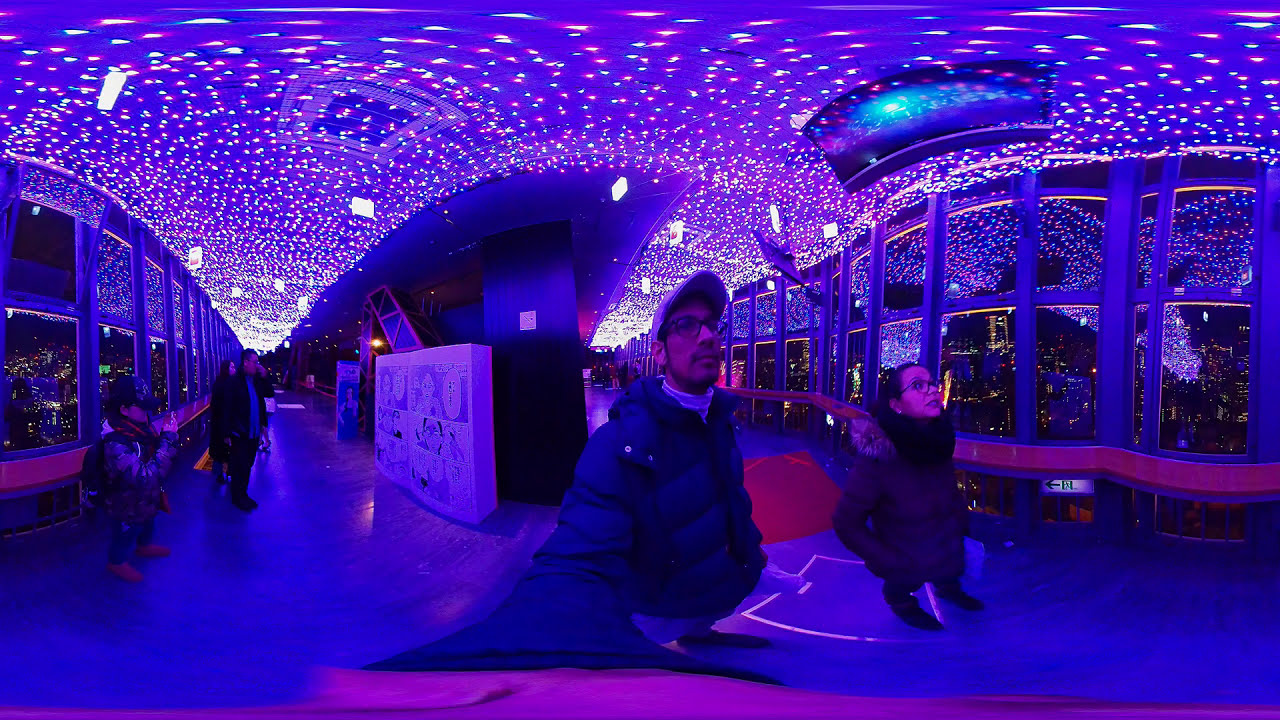The image depicts a crowded indoor art gallery or museum featuring a vibrant light display. Multicolored lights, from white to red and blue, cover the ceiling, creating a dazzling effect. In the center of the scene, a man with a white cap, glasses, and a beard, wearing a puffy blue jacket, is filming the event, possibly live streaming it. Beside him is a woman in a reddish winter coat with a furry hood and black scarf, also wearing glasses. Both are looking upwards, captivated by the light show above. The gallery space is divided, with windows on both the right and left sides and a central structure resembling an upside-down raft. Leaning against this structure is a large board covered in pictures. In the background, several people are visible, walking and observing the exhibit. On the far left, someone likely dressed in camouflage and a ball cap is taking a picture, adding to the lively ambiance of the scene.